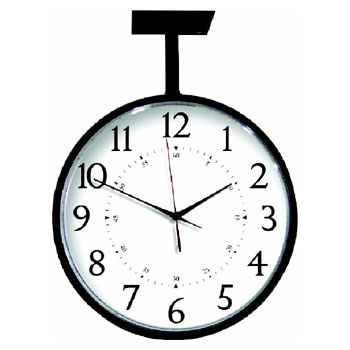The image features a clock suspended from the ceiling against a completely white background, giving it an isolated and minimalist appearance. The clock is characterized by a fusion of geometric shapes: a black square at the top and a rectangular body beneath it. The clock face displays a standard numerical arrangement with the numbers 1 to 12 in a circular formation, starting with 12 at the top and 6 at the bottom. 

The minute hand points at the 10-minute mark, the second hand is aligned with the 12, and the hour hand rests at the 2. Encircling the clock face are small dash marks denoting each minute, with bold triangular markers highlighting the key positions at 3, 6, 9, and 12 o'clock. The combination of these elements creates a cohesive and detailed representation of time.